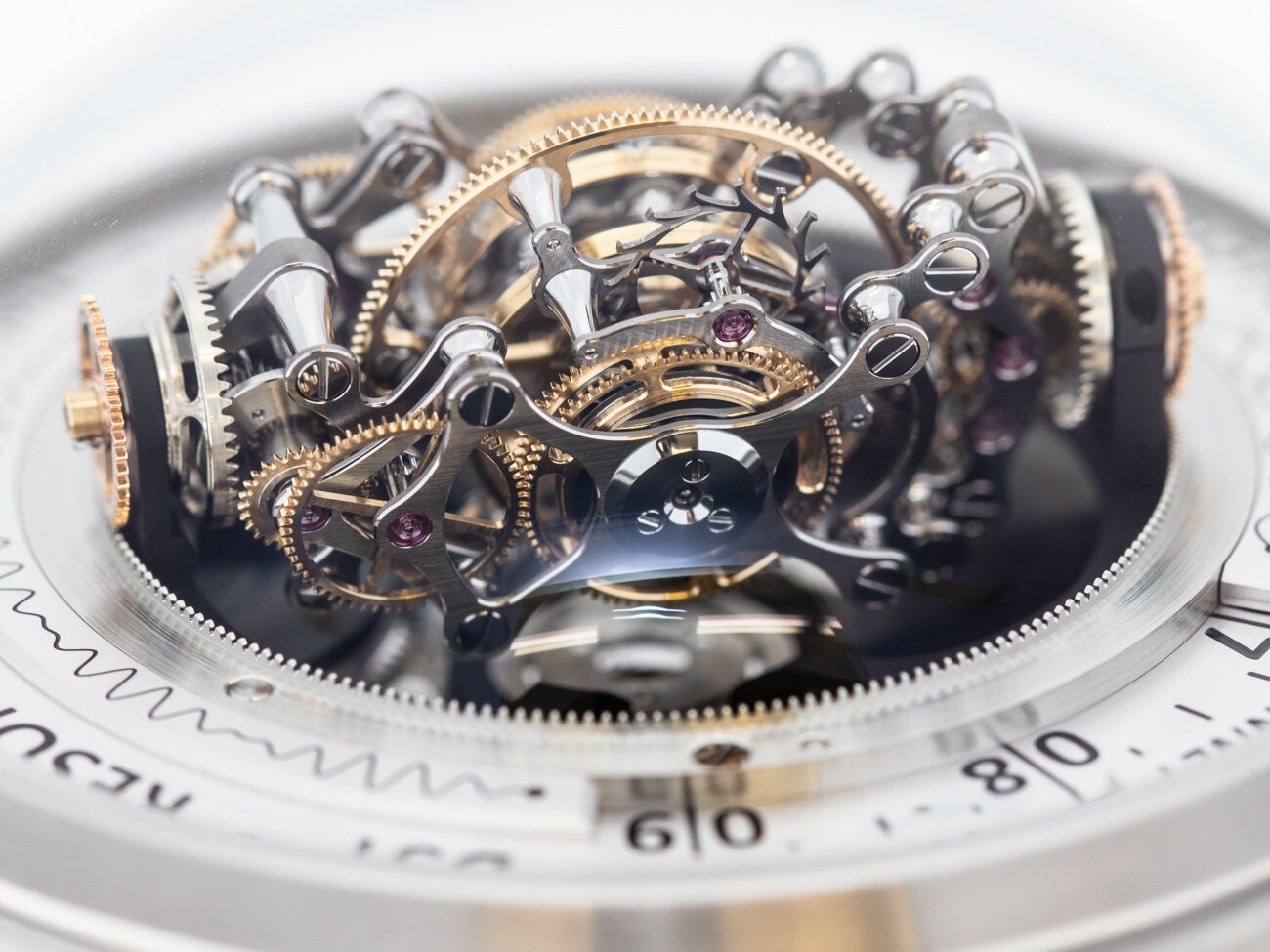This detailed photograph captures the intricate inner workings of a circular measurement tool, resembling a sophisticated combination lock. The silver dial prominently displays the numbers 60 and 80 at the lower portion, with number hashes and lines etched around its perimeter, echoing those of a clock face. The image is highly zoomed in, revealing an elaborate array of gears in the center. These gears range in size, with larger ones positioned centrally and progressively smaller ones extending outwards. The gears are crafted in both gold and silver hues, with flat head screws—some of which are lavender-colored—securing them in place. The screws vary in size, with larger ones on the exterior and smaller ones on the interior mechanisms. The largest gear, visible amidst the assembly, boasts over 500 finely cut teeth, while the smallest has over 200, highlighting the incredible precision and complexity of the device. The entire setup suggests a highly intricate mechanical design, much like that found in high-end watches or sophisticated engineering tools.